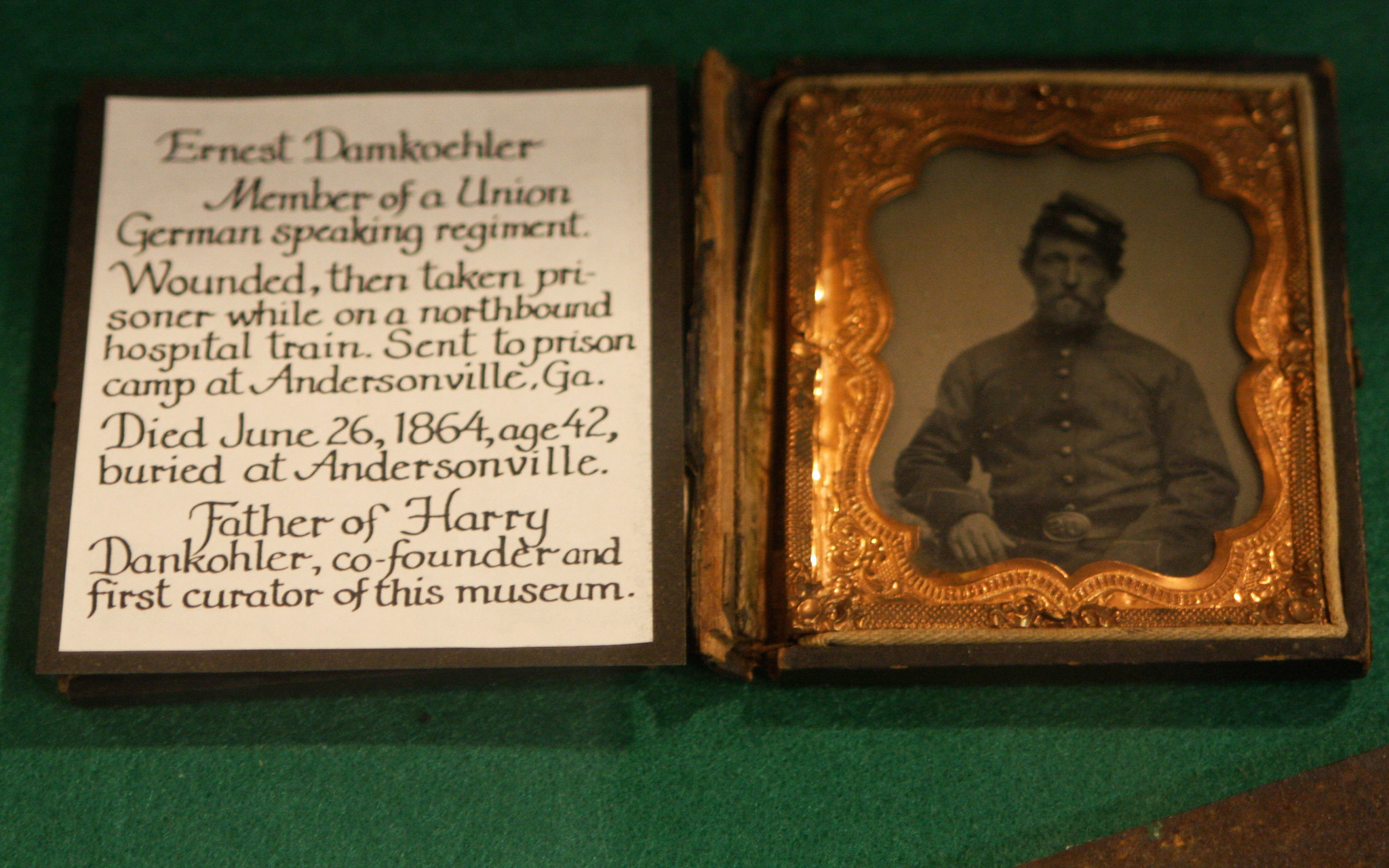The image showcases a rectangular photograph with a wider-than-tall aspect, resting on a green felt background. The main focus is an ornately framed black-and-white picture of a Civil War soldier in a dark uniform, identified as Ernest Damkohler, a member of a Union German-speaking regiment. The beautiful, embossed golden frame is open, with its top portion laying to the left. Positioned to the left of the photograph is an informative plaque with a brown border and white background with brown print. The plaque details that Ernest Damkohler was wounded and taken prisoner while on a northbound hospital train, subsequently sent to Andersonville prison camp in Georgia, where he died on June 26, 1864, at the age of 42. He was buried at Andersonville. Ernest was the father of Harry Damkohler, co-founder and first curator of the museum where this display is housed. The entire setup rests on the green felt, with a hint of a brown triangle shape in the lower right-hand corner, likely part of the table beneath.